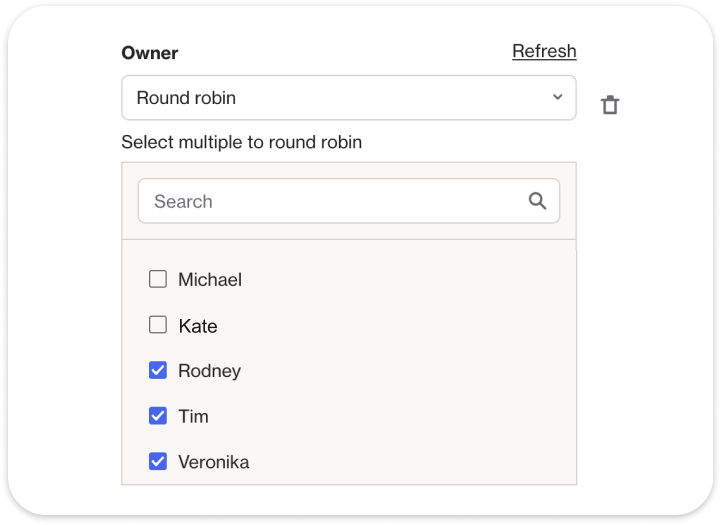The image features a white, square interface with rounded edges and a gray border. At the top of the interface is the word "Owner" in bold black letters. To the right of this, there is an underlined word "Refresh." Beneath these headers, a text box accompanied by a drop-down menu displays the text "Round Robin," with a trash can icon situated to its right.

Below this, the text "Select Multiple to Round Robin" is displayed. The middle section of the interface contains a gray square area with a search box at the top, featuring a magnifying glass icon. A gray line separates this section from the area below.

At the bottom, there are five checkboxes aligned on the left, each corresponding to a name on the right. The names, listed from top to bottom, are Michael, Kate, Rodney, Tim, and Veronica. The checkboxes next to Tim, Rodney, and Veronica are checked and highlighted in blue. The remainder of the interface consists of empty space.